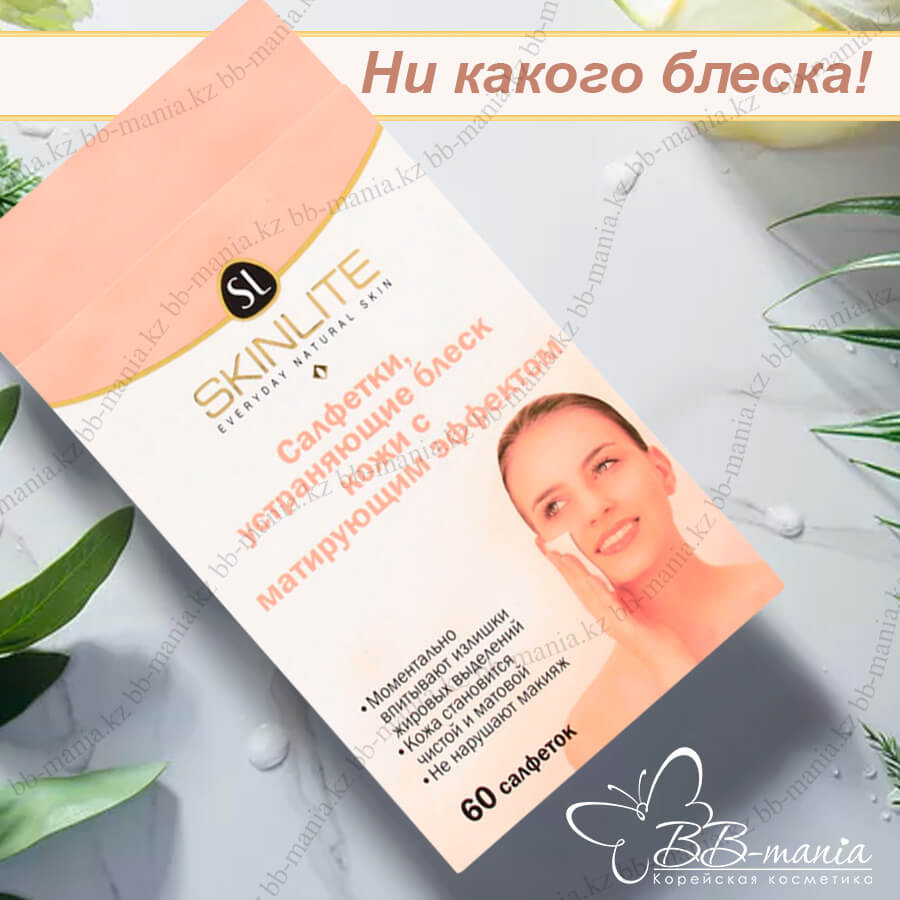This color image depicts a rectangular brochure for a skin care product, prominently featuring an image of a light-skinned woman smiling while touching her face with a facecloth. The background is mostly white, with green plant leaves extending from the edges, adding a touch of natural elegance. The brochure, angled from the top left to the bottom right within the square frame, has a peach-colored top section transitioning to white below. Central to the image is the branding "Skinlite," with a black "SL" logo above it, and the phrase "Everyday Natural Skin" in English. The skin care product, which appears to be a 60-pack of facecloths or makeup removers, is surrounded by additional text in a foreign language, possibly Russian, printed in dark pink and positioned at both the top of the brochure and on a banner behind it. The scene is clean, inviting, and stylish, effectively conveying the natural and everyday usability of the product.